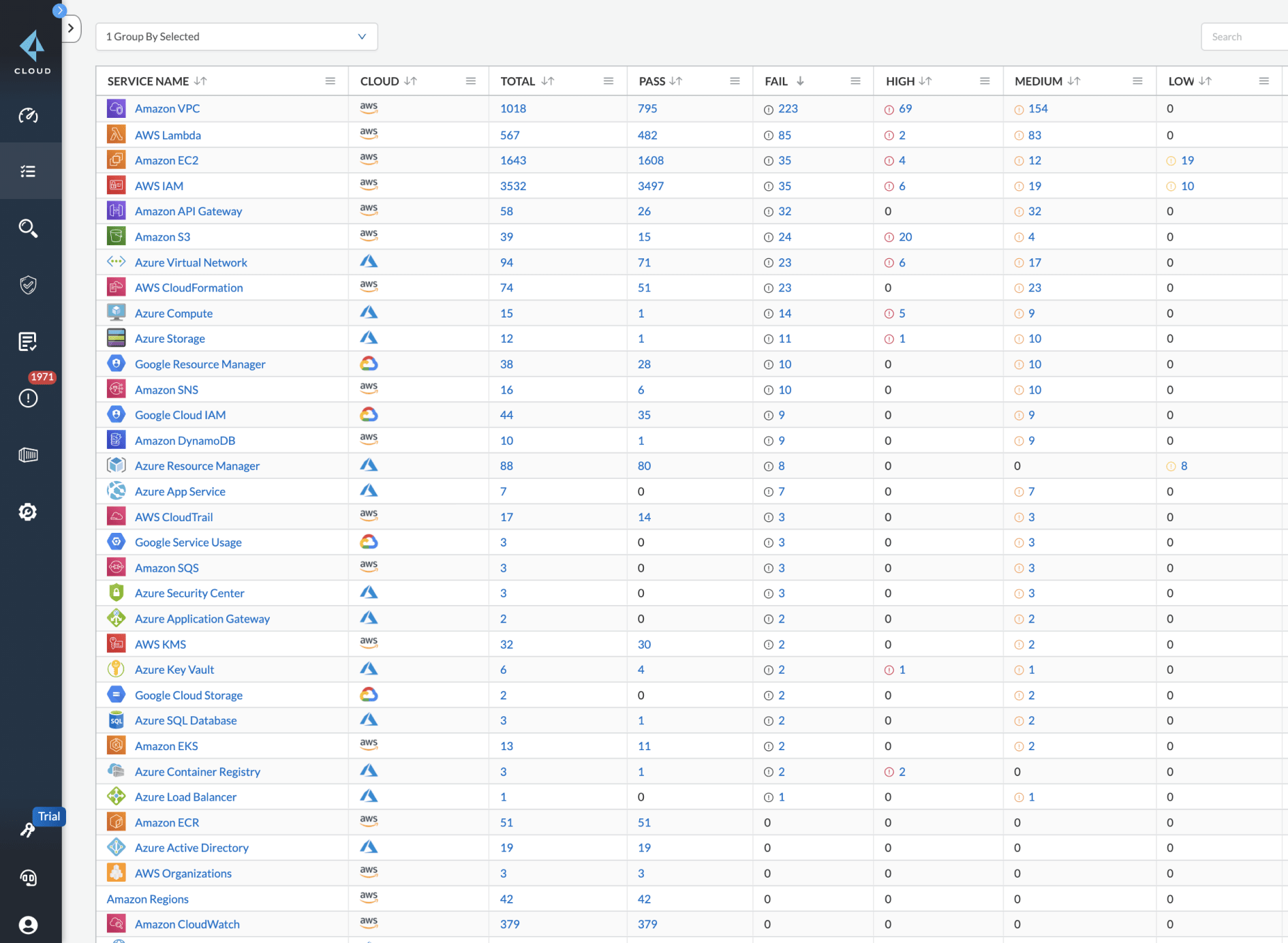This screenshot showcases a user interface with a primary focus on cloud services management. In the upper left-hand corner, the page is titled "Cloud," accompanied by a blue, angular icon directly above it. The interface features a consistent dark blue or black vertical border running along the left side. The main area of the screenshot is set against a gray background and is populated with several tables organized both horizontally and vertically.

These tables are delineated by various headers, including "Service Name," "Cloud," "Total," "Pass," "Fail," "High," "Medium," and "Low," providing a detailed breakdown of each service's performance and status. At the top left, there's an option labeled "Group by Selected," allowing for customized viewing of the data.

Prominent service names visible in the tables encompass a wide array of cloud services, such as Amazon VPC, AWS Lambda, Amazon EC2, AWS IAM, Amazon API Gateway, Amazon S3, Azure Virtual Network, AWS CloudFormation, Azure Compute, Azure Storage, Google Resource Manager, Amazon SNS, Google Cloud IAM, Amazon DynamoDB, Azure Resource Manager, Azure App Service, AWS CloudTrail, Google Service Usage, Amazon SQS, Azure Security Center, Azure Application Gateway, AWS KMS, Azure Key Vault, Google Cloud Storage, Azure SQL Database, Amazon EKS, Azure Container Registry, Azure Load Balancer, Amazon ECR, Azure Active Directory, AWS Organizations, Amazon Regions, and Amazon CloudWatch. 

Overall, the screenshot provides a comprehensive overview of various cloud services, facilitating easy monitoring and management.